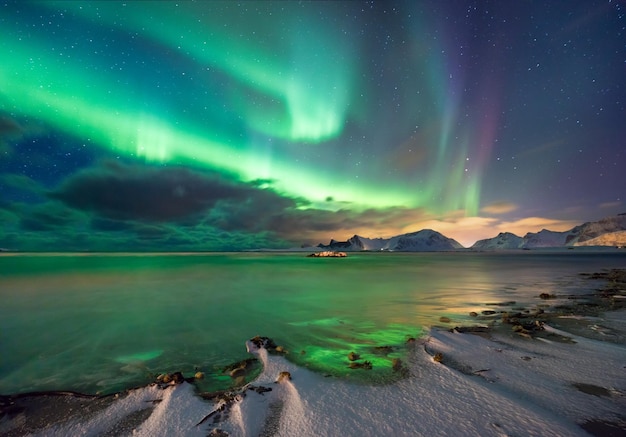The image depicts a stunning view of the Aurora Borealis with vivid, bright colors lighting up the night sky. The sky in the upper right corner is clear, showcasing a sprinkle of stars, while towards the bottom left, clouds form along the horizon. Predominantly, the auroras exhibit a bright green that fades into almost white hues and transitions into purplish tones as they move rightward. Snow-covered mountains are visible in the distance, adding a dramatic backdrop.

Below the auroras lies a body of water or possibly ice, its surface reflecting the vibrant greens and purples in a supernatural glow. At the very bottom right, the shore of this waterbody can be seen, covered either in snow or white sand, with the auroral lights casting an ethereal tint over it. The entire scene, with its contrasting elements and spectral lights, captures the mystical essence of nature at night.